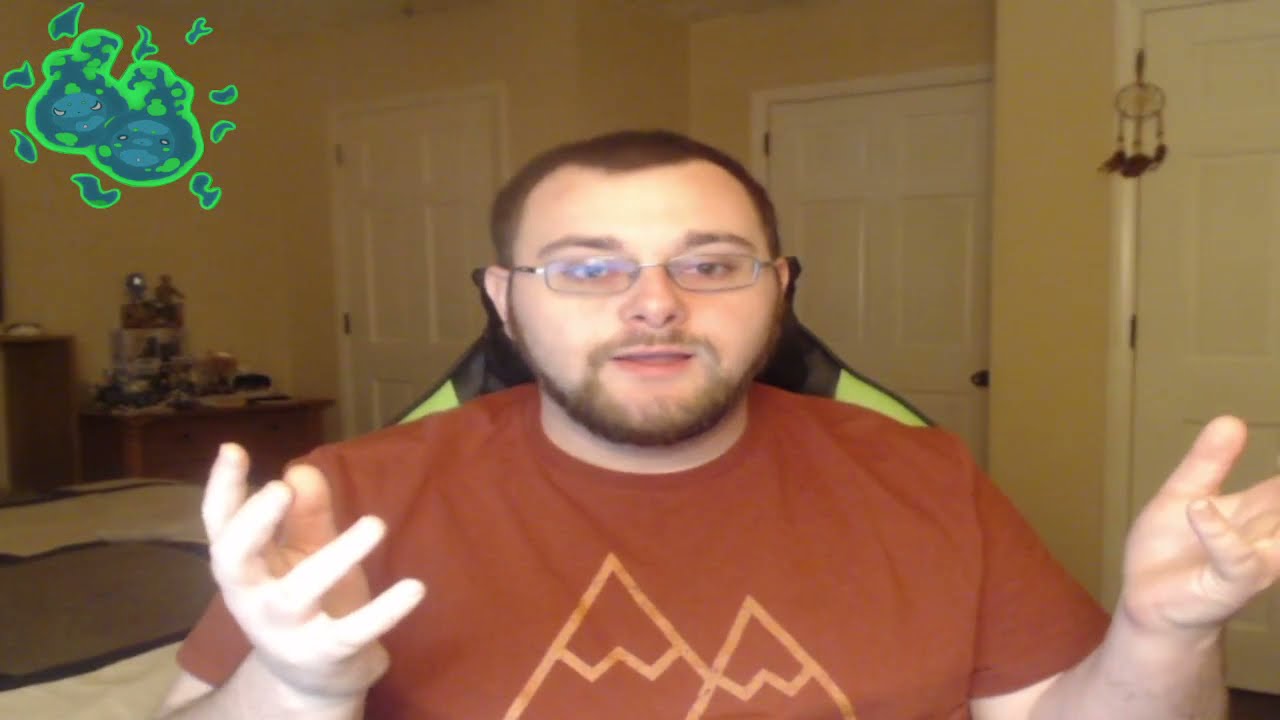In the image, a man with a prominent receding hairline and very short hair is sitting in a black and green gaming chair. He is wearing a brown short-sleeved t-shirt featuring two light brown mountains, each with a 'W' symbolizing snow or ice on top. The man has oval-shaped glasses, a mustache, and a full beard, with his hands raised and slightly bent as if he is mid-conversation, his face expectant and mouth slightly open. 

To the right of the man, there is a room's door adorned with an Indian dream catcher. The background reveals a mixture of yellow and white walls with another white door with a black handle, possibly open. Adjacent to the wall is a nightstand cluttered with objects. Furthermore, there's a bed positioned against a brown headboard with a white bedspread featuring a large brown block in the center. In the top left corner of the image, a stylized blue and lime green logo, resembling two fish faces or raindrops, is visible.